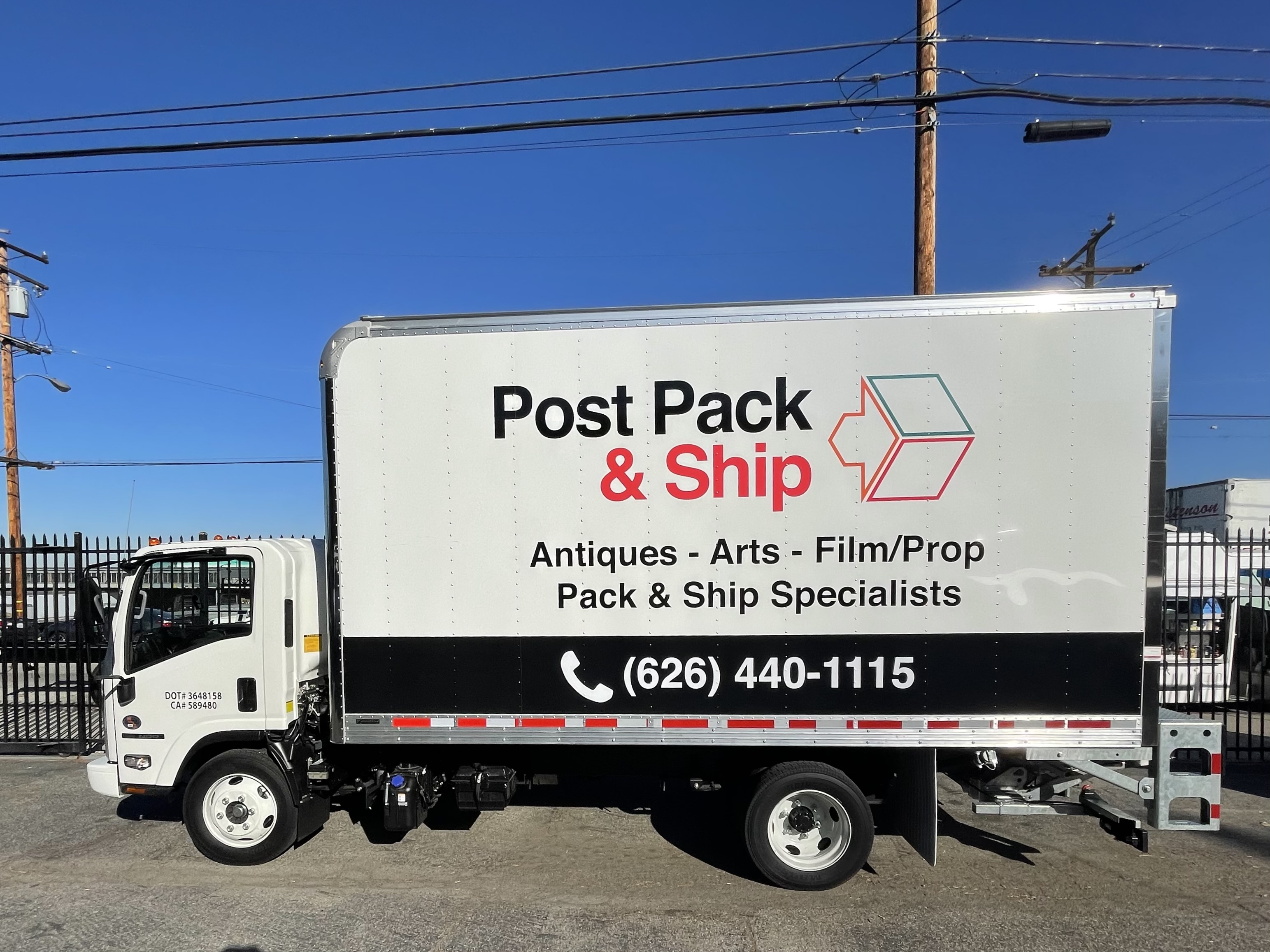The image depicts a box truck, specifically a small delivery truck, parked on a gray asphalt surface that appears to be a parking lot. The vehicle is primarily white, featuring a black border along the bottom side panel. The truck has a compact, boxy design typical of delivery vehicles smaller than full-sized interstate tractor-trailers but larger than passenger vehicles. On the side of the truck, the following text is prominently displayed: "Post-Pack and Ship" in black, with "Post," "and," and "Ship" in red. There is also a red and blue icon resembling a box with an arrow next to this text. Below this, the truck advertises services such as "Antiques," "Arts," "Film Prop," and "Pack and Ship Specialists" in black text. The black border beneath this text features a white phone number alongside a phone icon.

The truck is positioned in front of a black wrought iron fence, which separates the parking area from a backdrop of buildings and a utility pole. The scene is characteristic of an urban setting with typical infrastructure and commercial deliveries.